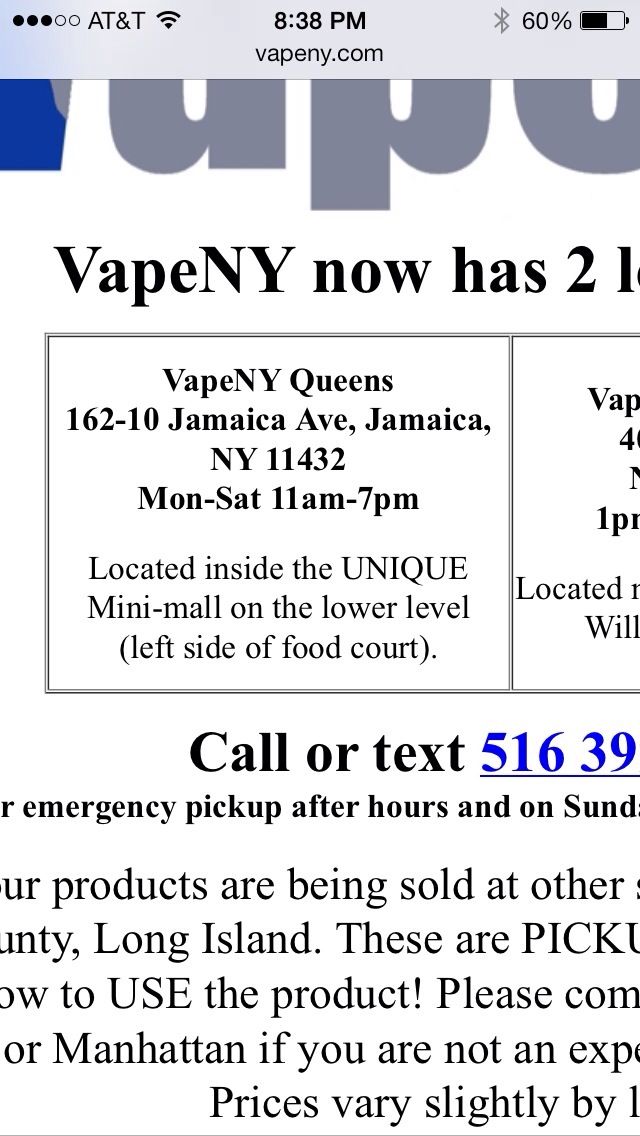The image is a screenshot from an iPhone displaying a webpage for a vape shop in New York. The phone's status bar shows it’s 8:38 PM, connected to AT&T with Wi-Fi, Bluetooth enabled, and 60% battery. The webpage URL is partially visible as "VAPenny.com." The main content reveals some details about the vape shop: “VAPenny Queens, 162-10 Jamaica Avenue, Jamaica, NY 11432,” with operating hours from Monday to Saturday, 11 AM to 7 PM. It’s located inside the UNIQA Mini Mall on the lower level, beside the food court. The primary text is in black against a white background, with additional information partially cut off, mentioning words like "emergency pickup after hours," "Sunday," "products sold at other," "Long Island," "how to use the product," and "Manhattan if you are not an." There’s also a blue underlined phone number starting with 516 for call or text. The zoomed-in nature of the screenshot makes much of the text difficult to read, leaving sections obscured or cut off.